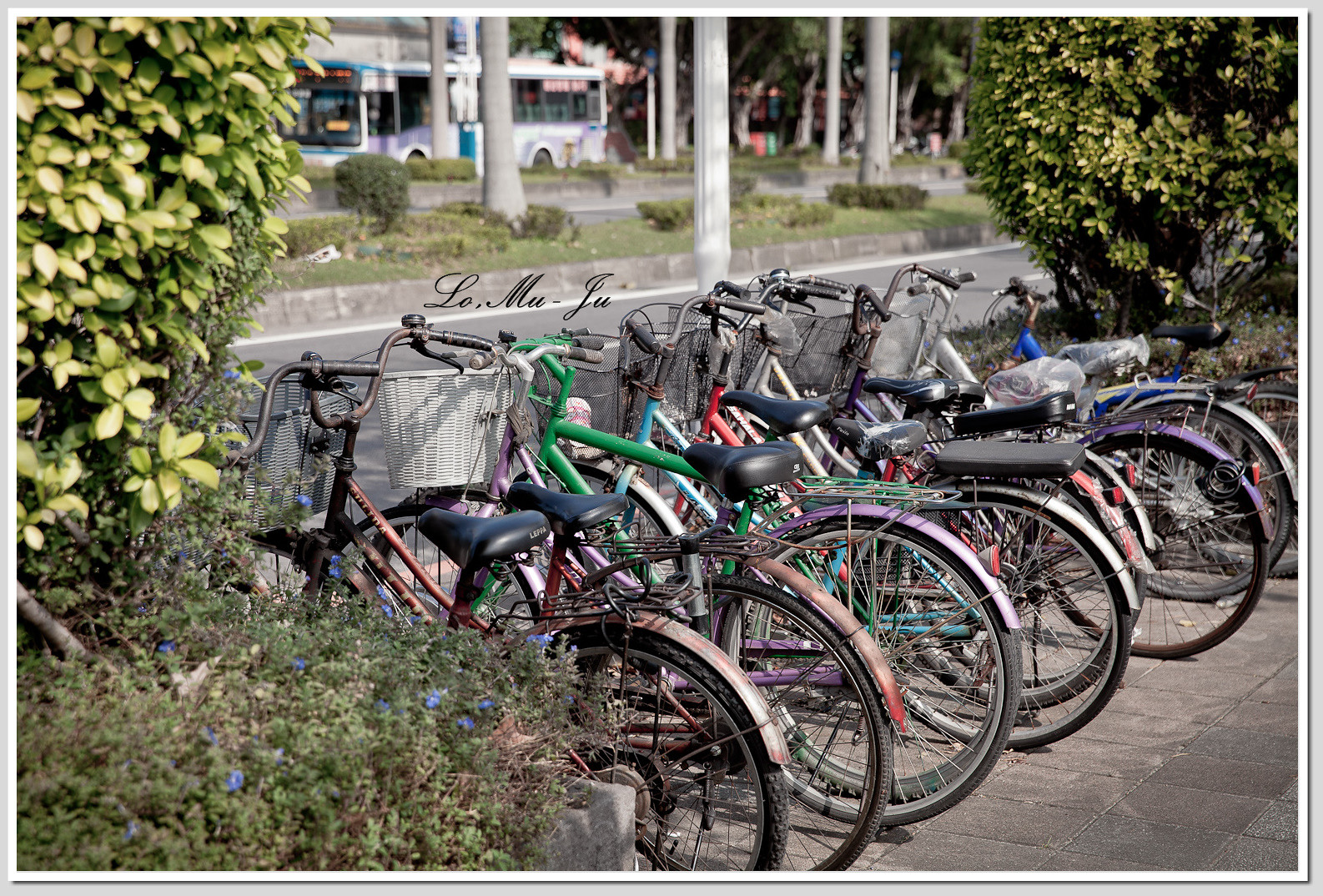The colour photograph, presented in landscape orientation, features a two-tone frame with a white bezel hugging the photo and a light grey outer bezel. Dominating the composition is a series of nine or ten bicycles, front-facing into a bike rack, their rear wheels closest to the viewer, extending from the front left towards the back right of the image. The bikes come in varying hues, including reddish silver, purple, green, blue, reddish-orange, white, and grey, with the purple one sporting a distinctive white wicker basket. Each bike has a platform behind the seat for cargo and identical baskets, save for the one exception. 

Centrally, though slightly off to the left, there is italicized text that reads, "Lo-mu-jo," albeit somewhat challenging to decipher. 

To the left and right of the bicycles are tall shrubs and bushes. The one on the left has an assortment of blue flowers, while the others have dark green and yellow foliage. Behind the bikes and their handlebars, a street scene unfolds in the background. Prominent details include a bus moving leftward, tall trees with light grey and white trunks, and a white utility pole ascending beyond the frame. The scene captures the blend of urban environment and nature, providing depth and context to the main focal point—the colorful line-up of bicycles.